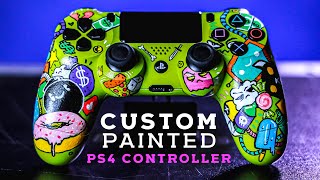The image depicts a horizontally oriented, full-color photograph taken indoors, showcasing a highly customized PS4 video game controller. The background is divided into distinct sections: the top third features a solid bright blue color, followed by a white strip, and the bottom two-thirds appear to be a brownish, textured surface, likely resembling a countertop. There's printed text at the bottom center of the image in white and purple that reads "custom painted PS4 controller."

The focal point of the photograph, a PS4 controller, is vividly painted in a neon green base color. Various cartoonish and animated images are intricately depicted across its surface, adding a unique and playful touch. On the lower left handle, a dripping pink donut is visible, alongside a blue sack of money with a white dollar sign. The right side under the knob showcases a pink Pac-Man ghost and a blue popsicle. Additionally, a slice of pepperoni pizza is illustrated under the left knob. Other whimsical elements include green dollar bills, a liquor bottle with a purple label featuring a white skull, a silver sword, and a white bone. The center of the controller displays two black circular buttons below a digital screen, which currently shows no display.